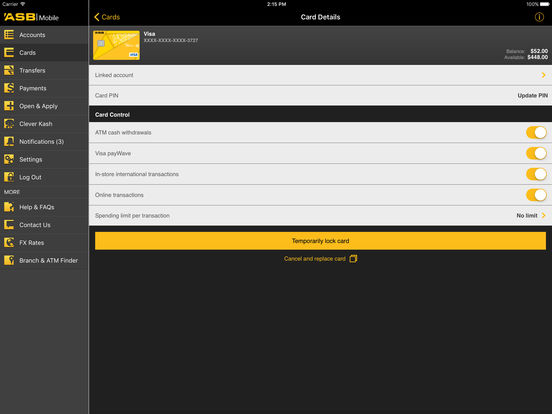The image showcases the mobile interface of an ASB banking application. Dominating the top-left corner of the screen, the recognizable yellow ASB mobile logo is prominently displayed. Below or beside this logo, a neatly organized list of functional buttons with yellow icons aligns vertically. These icons represent different features in the following order:

1. Menu icon labeled 'Accounts'
2. Credit card icon labeled 'Cards'
3. Two boxes with arrows indicating 'Transfers'
4. Dollar icon labeled 'Payments'
5. Plus icon labeled 'Open and Apply'
6. Alien icon labeled 'Clever Cash'
7. Bell icon labeled 'Notifications' followed by the number (3)
8. Gear icon labeled 'Settings'
9. Lock icon labeled 'Log Out'
10. Text saying 'More' followed by:
    - Question mark icon labeled 'Help and FAQs'
    - Message icon labeled 'Contact Us'
    - Earth icon labeled 'FX Rates'
    - Location icon labeled 'Branch and ATM Finder'

To the right, a larger detail-focused section is visible. A prominent black banner at the top reads 'Card Details,' noting the current time as 2:15. Beneath this banner lies a gray bar prominently featuring a mock-up of a yellow Visa card, partially censored, displaying 'XXX, XXX, XXX 3727'. To the right of the card, it shows 'Balance: $52' and 'Available: $448'.

Further down, two white buttons offer functionality for 'Link to Account' and 'Card Pin', with an 'Update Pin' button adjacent to these options. Following this, a black bar titled 'Card Control' presents more card management options, including:

- ATM Cash Withdrawals
- Visa PayWave
- In-Store International Transactions
- Online Transactions
- Spending Limit per Transaction

Each of the first four options features a slide switch on the right, all of which are activated. The last option indicates 'No Limit' accompanied by an arrow.

At the very bottom, a yellow button offers the option to 'Temporary Lock Card', while yellow text provides an option to 'Cancel and Replace Card'.